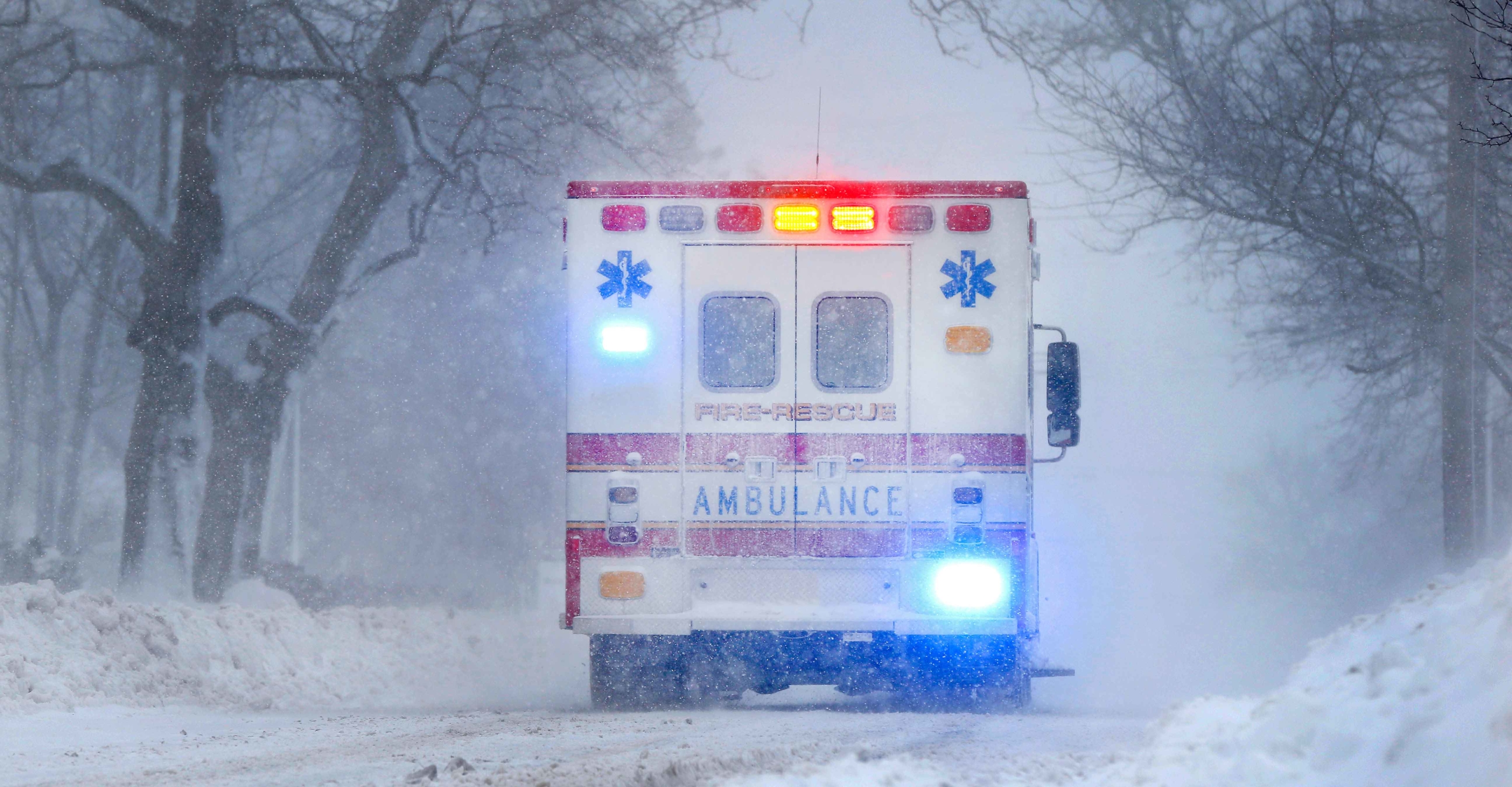This is a full-color photograph taken outdoors during the day, showcasing a snowy winter scene obscured by a heavy snowstorm. The horizontal image prominently features an ambulance driving away from the camera on a snow-covered road. The sky is gray, and falling snow creates a misty backdrop, adding to the sense of harsh weather conditions.

The ambulance, adorned with bright, flashing lights, has blue lights in its upper and lower left corners and two orange lights along the top rear. The vehicle is primarily white with red stripes and clearly marked with "Fire Rescue" in orange and "Ambulance" in blue text on its back. Additionally, blue ambulance symbols are visible on its left and right sides.

The road is blanketed in thick snow, with visible tracks suggesting limited visibility of underlying dirt. Piles of snow line both sides of the road, and the trees flanking the path are barren and heavily coated with snow, creating a canopy-like effect. The vehicle's slow progression through the snowstorm conveys a sense of urgency and caution.